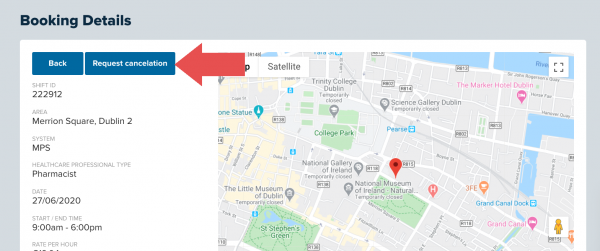The image depicts a web page focused on booking details, framed by a light bluish-purple border. At the top left corner, the title "Booking Details" is prominently displayed. Just below this, there is a button labeled "Back" alongside another button marked "Request Cancellation," indicated with an arrow pointing towards it.

The main contents of the page include specific booking information:

- **Shift ID:** 222912
- **Location:** Merlin Square, Dublin 2
- **Role:** MPS Pharmacist
- **Date:** 27th June 2020
- **Start Time:** 9:06 AM
- **End Time:** 6:00 PM

To the right of these details, a map is displayed, featuring a pin dropped near the National Museum of Ireland. This map highlights several blocks around the museum, illustrating local tourist destinations, parks, and harbors, suggesting a potential booking at or near the museum. The individual seems to be in the process of canceling this booking request.